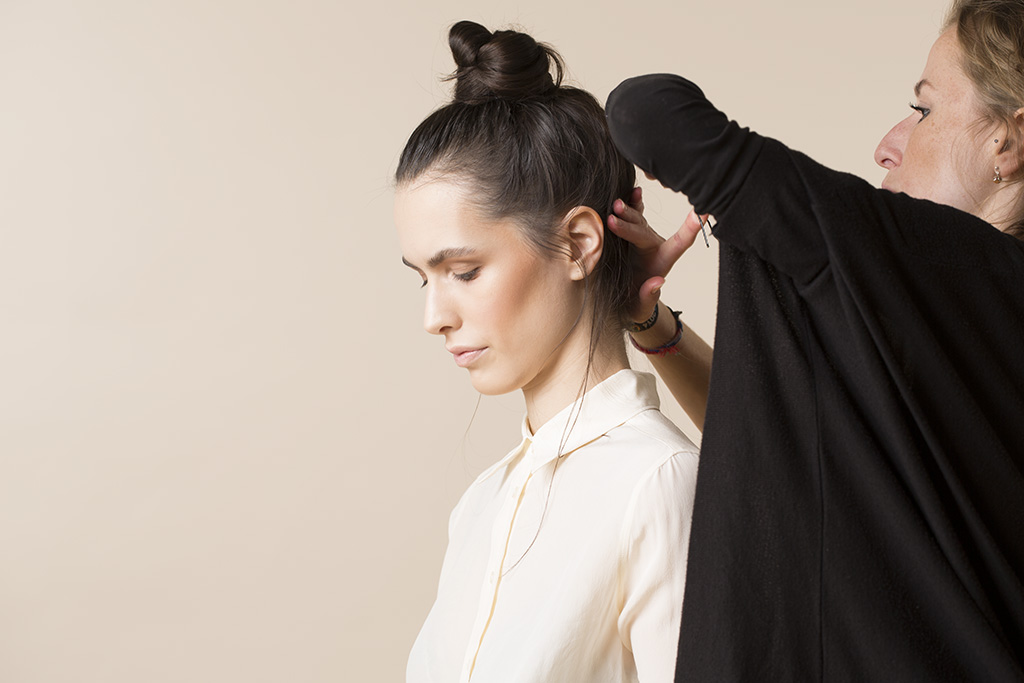The photograph captures an intimate styling moment between two women against a tan backdrop. At the center, a woman with fair skin has her brown hair twisted up in a bun. She wears a cream-colored button-down blouse and has makeup applied to her face, giving her a polished look. Her eyes are gently closed, and she appears to be looking down towards her lap. Standing beside her to the right, the hairstylist is a white woman with dark blonde, sandy hair. She wears a black long-sleeve shirt and gold earring. With both hands focused on shaping the bun, one holding a device unseen in the photo, the stylist's elbow is bent, indicating concentration and care in her work. Her partial profile is visible, showing her attentiveness to the task. The background is a seamless tan color, adding warmth and highlighting the serene moment.